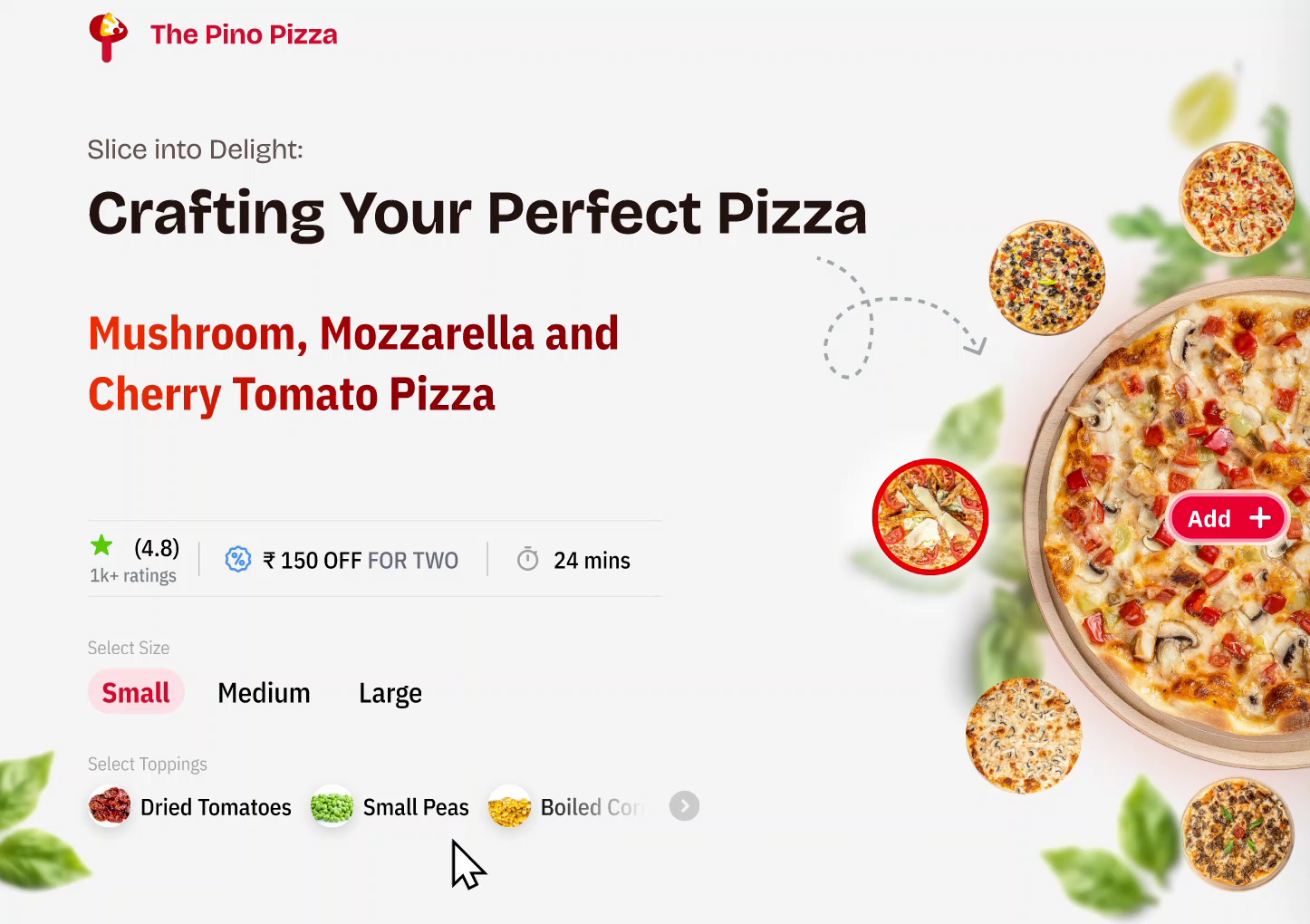This image is an advertisement for Pino Pizza, showcasing their enticing offer to craft your perfect pizza. The largest text prominently states "Crafting Your Perfect Pizza" in bold black font. On the far right side, a large, delectable pizza photo is surrounded by five smaller images of various pizzas, providing a tantalizing visual feast. The background, slightly blurred, features fresh basil leaves, hinting at the quality ingredients used by the pizzeria.

Beneath the main headline, the selected pizza is a mouth-watering combination of mushrooms, mozzarella, and cherry tomatoes, written in a striking dark red font. Just below this is the restaurant's impressive rating of 4.8 stars, illustrated with green stars. The interface allows customers to choose their desired pizza size—small, medium, or large. The current selection is small, highlighted in pink with the font in red, emphasizing the customization options Pino Pizza offers.